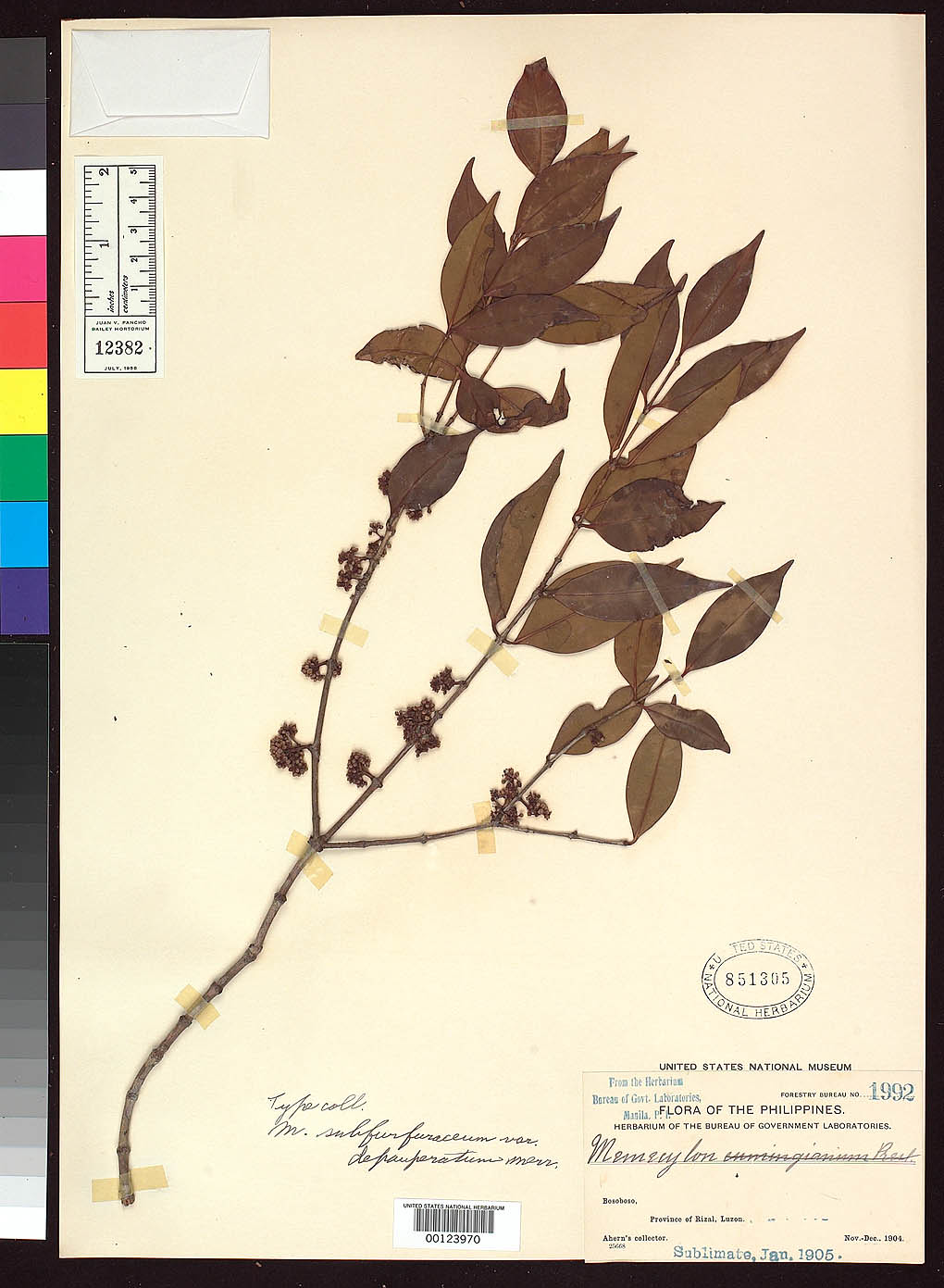The image depicts a preserved botanical specimen affixed to a yellowing, beige document. This document, marked with the number 851305 and stamped "United States National Herbarium," features a pressed twig with several branches, leaves, and potentially some dried flowers, secured with visible tape. The plant, labeled illegibly in black ink, angles from the lower left to the upper right corner. Handwritten cursive inscriptions accompany multiple printed texts.

A small envelope is taped to the upper left corner, possibly for seeds, alongside a vertically oriented paper ruler for size reference, displaying measurements in inches and centimeters. There is also a color swatch on the left side, exhibiting shades from gray to pink, yellow, green, dark blue, black, and white, likely for color comparison.

The document bears additional labels and stamps: a sticker with a scan code reading 00123970, "United States National Herbarium," and "Ahern's Collector" above an illegible number. Further inscriptions include "Forestry Bureau number 1992," "Province of Rizal, Luzon," dated "November-December 1904" with "sublimate January 1905" beneath it. The scene is framed by a black border, except for the left side, which is edged with vibrant squares of various colors.